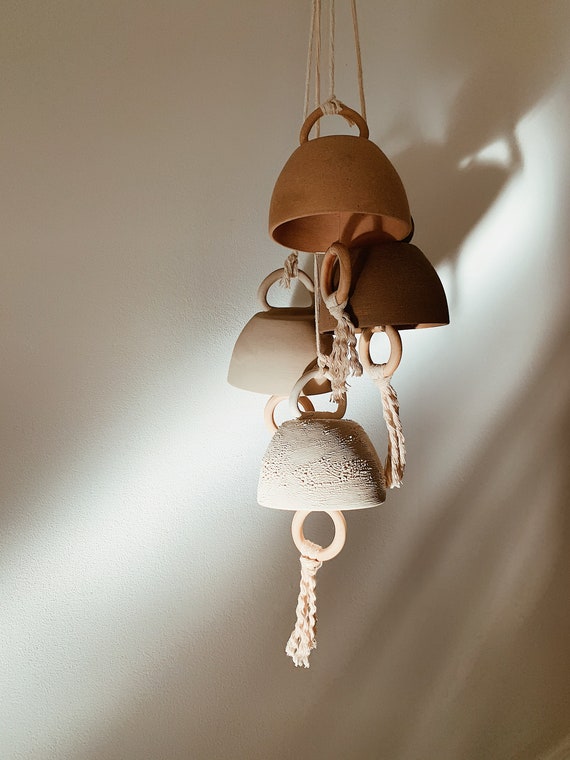The photograph showcases a creative arrangement of four clay bowls hanging from thick white strings against a light gray wall, with sunlight casting intricate shadows. Each bowl features a prominent handle, allowing them to be securely tied and suspended upside down at varying heights, creating an intertwined, bell-like formation. The topmost bowl is a large, orangish-tan color, followed by a dark brown bowl. Beneath these, there are two lighter-colored bowls: one ivory and the bottom-most one being white with distinctive bumpy textures, possibly floral engravings. Each bowl has a string running through its center, connecting to a color-coordinated ring, from which a tassel-like rope hangs. The entire assembly emits an aura reminiscent of wind chimes, with the interplay of colors and textures adding a unique charm to the scene.